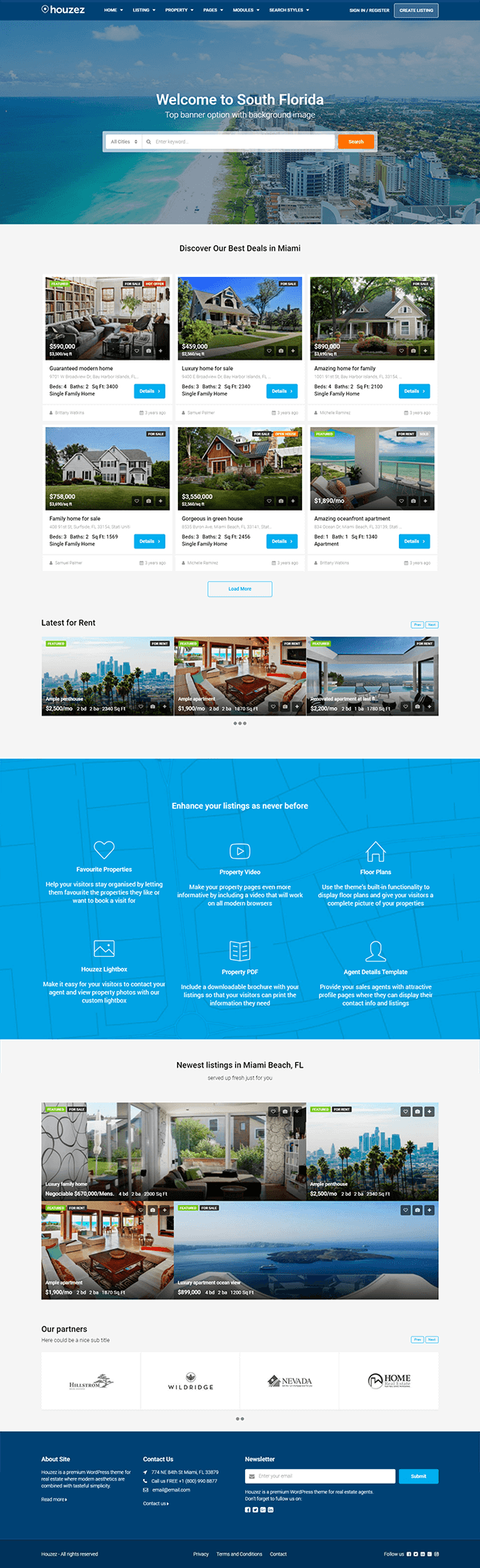This image appears to be a screenshot from a real estate website named "HOUZEZ." At the top, there's a welcoming message: "Welcome to South Florida," accompanied by a prominent banner. The background image of this banner showcases beautiful beachfront properties, capturing the essence of South Florida's coastal living.

Beneath the welcoming banner, bold text invites users to: "Discover our best deals in Miami." This is followed by a series of thumbnail listings featuring various Miami properties. Though the text on these listings is difficult to read, it appears that many of them are high-end, potentially with prices reaching seven figures.

Further down, the caption "Latest for Rent" suggests a section dedicated to rental properties. Another segment is visible below, bearing the text: "Enhance your listings as never before." This section seems to cater specifically to realtors, offering tools and features to improve property listings. These features include symbols like a heart (favorites), a play button (video preparations), a house icon (floor plans), a book (property PDFs), and a person silhouette (agent detail templates).

Continuing down the page, there are additional property listings with the heading: "Newest listings in Miami, Florida," highlighting the latest additions from the Miami area.

At the bottom of the page, a section titled "Our partners" lists various affiliated businesses, indicating strong collaboration networks within the real estate market.